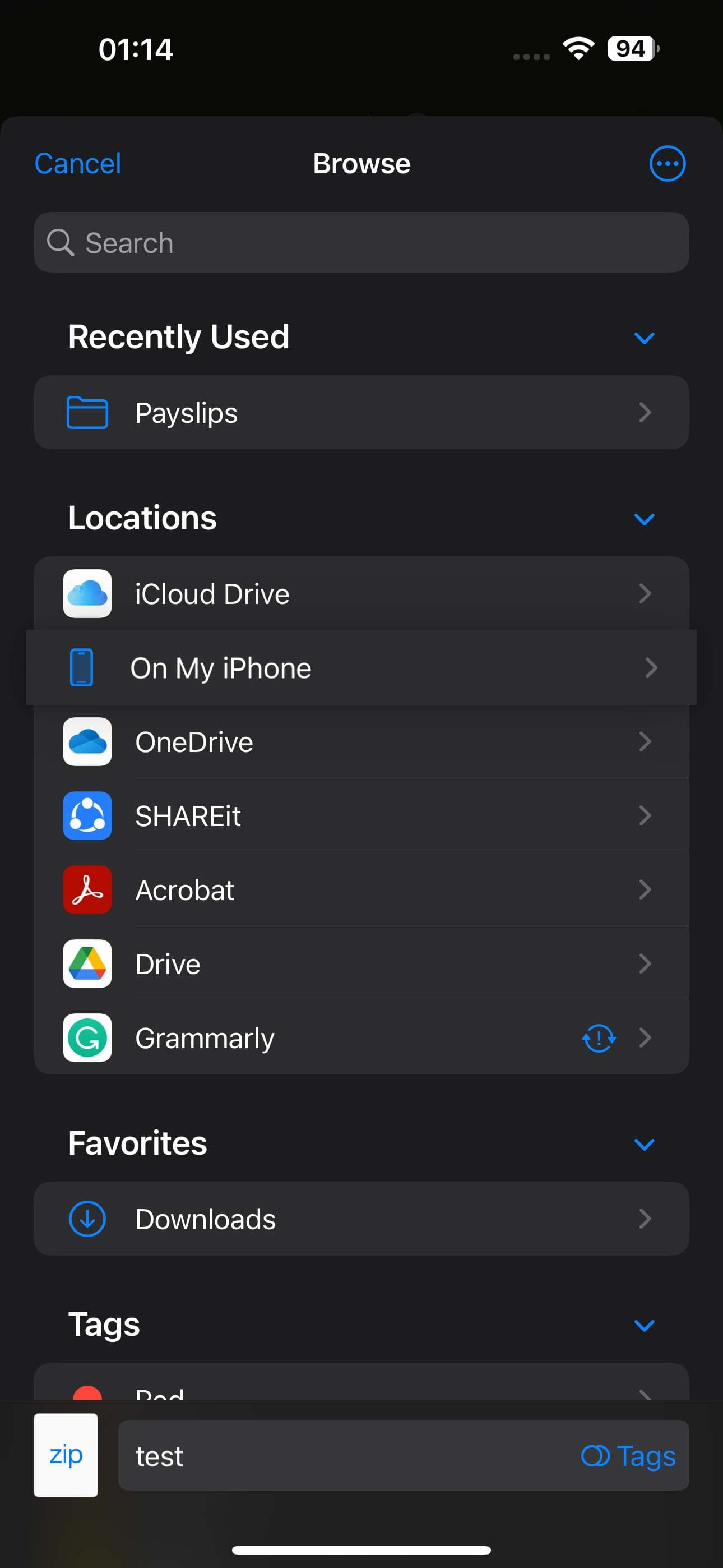The image displays a detailed view of a digital interface, likely from a mobile device or application. At the top left corner, it shows the time "01:14". Directly to the right of the time, there are four small grey dots aligned horizontally. Following the dots are icons for Wi-Fi and battery status, the latter displaying "94M Black".

Beneath this top row, there is a slightly grey line containing three elements: "Cancel" written in blue, "Browse" in bold white letters, and an outlined circle with three horizontal dots within it.

Below this line is a dark grey rectangular search bar featuring a magnifying glass icon and the word "Search". 

Next, in bold white letters, there is a heading that reads "Recently Used", accompanied by a down arrow on its right side.

Further down, there is a grey rectangular section displaying a folder icon followed by the label "Payslips" and a right arrow. 

Following this, there is another section with the heading "Locations" in bold letters, along with a down arrow. This section lists several icons with corresponding labels and right arrows: 
- iCloud Drive icon
- On My iPhone icon
- OneDrive icon
- Share It icon
- Acrobat icon